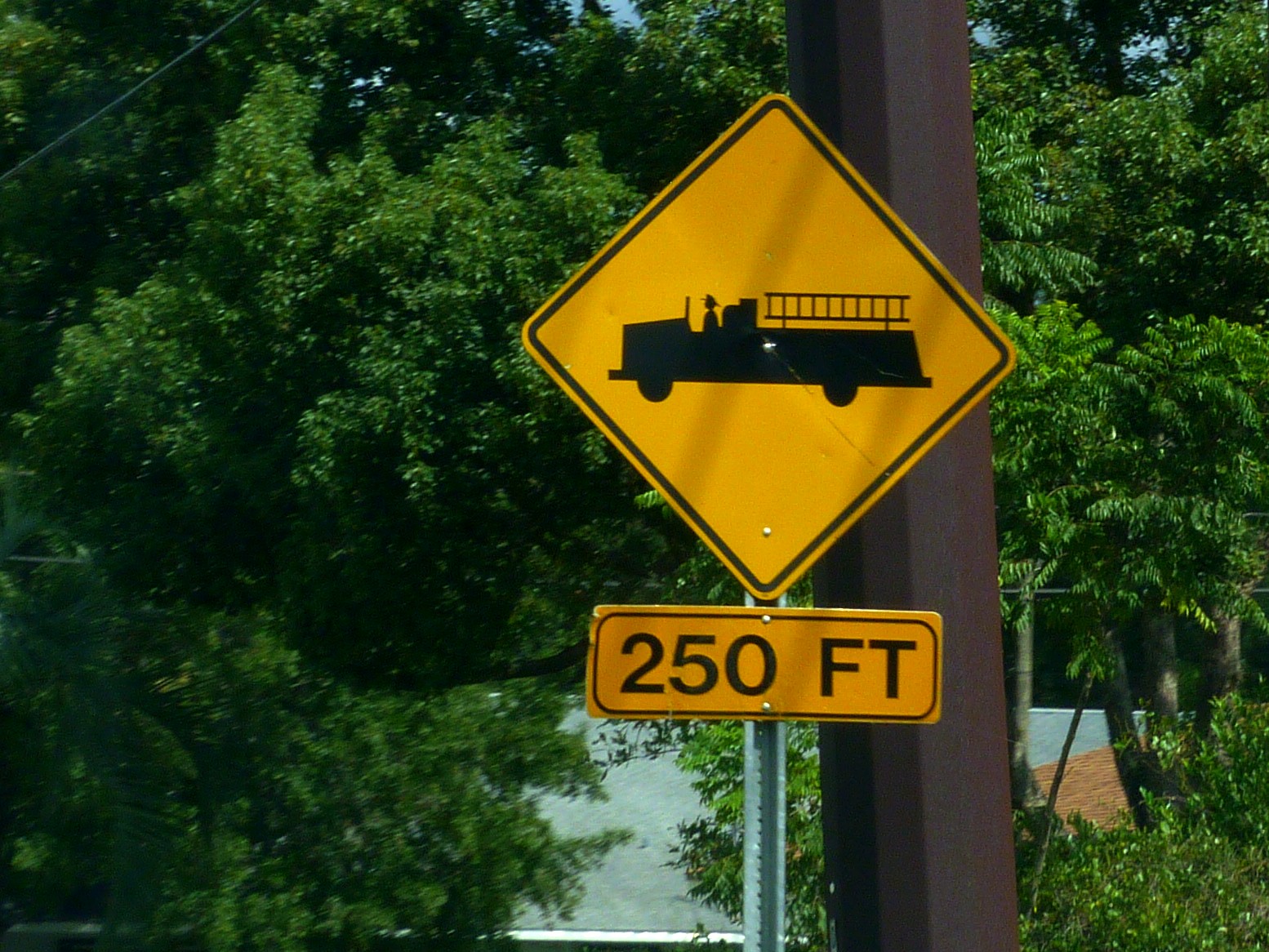The image features a yellowish-orange diamond-shaped caution sign mounted on a metallic pole. On the sign, there is a black silhouette of a fire truck, clearly showing a driver wearing a hat in the driver's seat and a ladder extending horizontally from the back of the truck. Beneath this main caution sign, there is a smaller yellow rectangular sign stating "250 FT." In the background, a large black pole is visible amidst dense vegetation, including numerous trees and their trunks on the right-hand side. At the bottom, there is a bluish-gray area that appears to be a lake, accompanied by a dirt patch next to it.